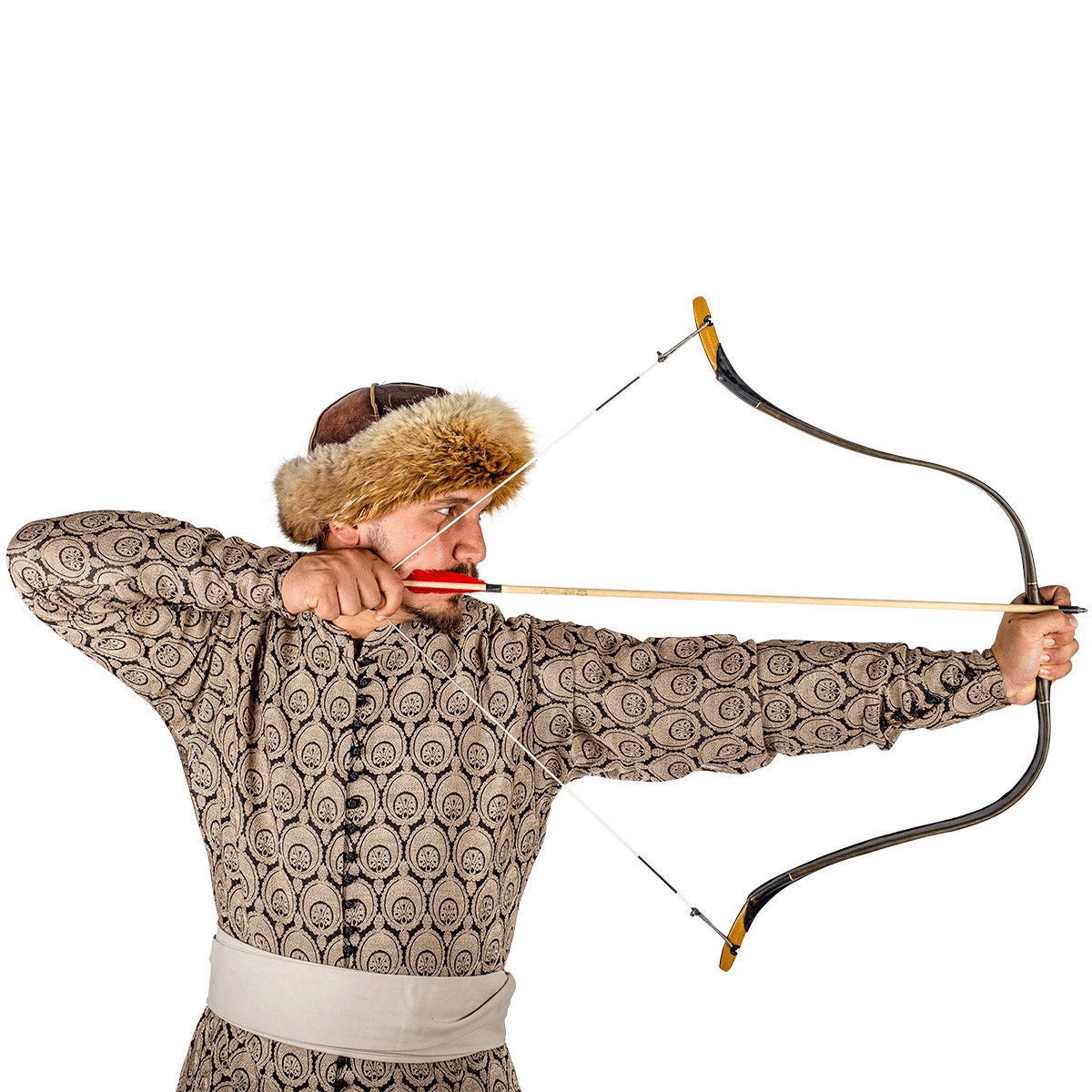A white-background image showcases a poised archer with remarkable detail. The archer, a Caucasian male, sports a meticulously groomed goatee and mustache. His intense gaze complements his focused posture. He dons a fur-rimmed hat with a brown top, adding an element of rugged charm to his medieval-inspired attire. His dark taupe, long-sleeved tunic is adorned with repeated circular patterns, each resembling an oval with an inner circle, exuding a sense of historical authenticity. Around his waist, a taupe-colored sash cinches his ensemble. The archer's black bow is fully drawn, the tension palpable as the arrow points decisively to the right, ready to be unleashed.